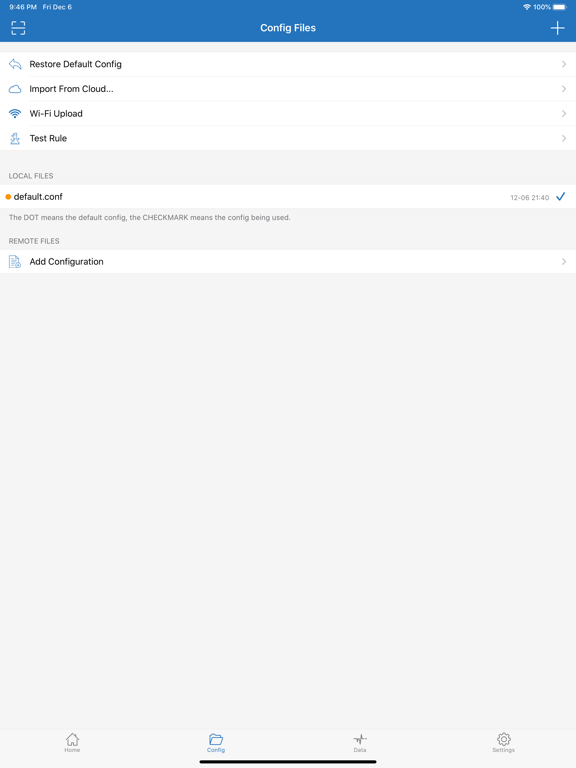Screenshot depicting a software interface:

At the top of the screen, you can see a blue rectangle with white text indicating the current time as "9:46 p.m." on "Fri Dec 6." Toward the left upper corner, there is a square icon with a line through it which is labeled as "config files." 

In the upper right-hand corner, status indicators are displayed: a Wi-Fi symbol, "100%" battery charge icon filled in white, and a plus sign.

Below these indicators, there is a leftward-pointing arrow labeled "restore default config." Adjacent to this is a cloud icon featuring the text "import from cloud..." There is also a Wi-Fi signal icon labeled "Wi-Fi upload."

Further down, there is an icon resembling a stick figure with the label "test rule." Beneath this section, an area marked "Local Files" contains the text "default Conf" with an orange dot beside it.

The rest of the interface background is gray, with a button at the bottom labeled "add configuration."